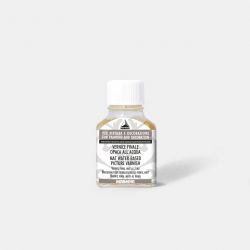The image depicts a small, travel-sized bottle with a white cylindrical cap. The bottle is transparent and appears to hold a liquid. It features a white label with a gray text box containing white letters, though the text is blurry and difficult to decipher. The label also includes black text, likely listing the ingredients or a description. The bottle is square-shaped and sits against a predominantly white background, which takes up the majority of the space in the image. The background has subtle gray tones, adding a slight contrast to the scene. Given the bottle's small size and detailed labeling, it seems to be intended for a specific purpose, possibly touch-up work or an application requiring a minimal amount of liquid.